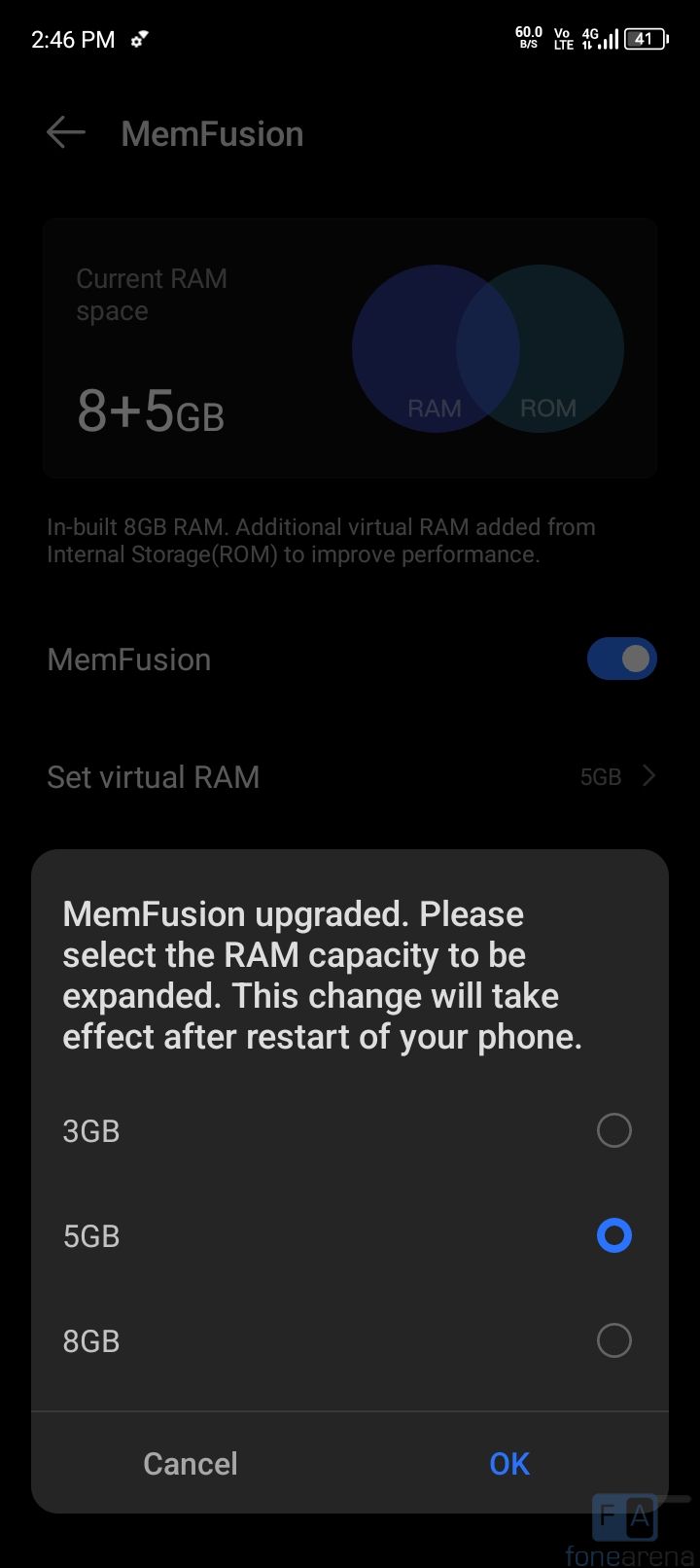The image displays a smartphone interface with a black background at 2:46 p.m. Prominently featured is a notification panel detailing memory management options:

1. An informational section outlines current RAM configuration with a left-pointing arrow labeled "Mem Fusion," indicating "Current RAM Space: 8 + 5 gigabytes."
2. Below this, a large blue circle labeled "RAM" and a gray circle labeled "ROM" explain, "Inbuilt 8GB RAM with an additional 5GB virtual RAM added from internal storage (ROM) to improve performance."
3. Another "Mem Fusion" label appears with a blue toggle switch, offering the option to "Set Virtual RAM" at 5 gigabytes. 
4. A right arrow and a bordered box read, "Mem Fusion upgraded. Please select the RAM capacity to be expanded. This change will take effect after the restart of your phone."
5. Within the box, in white print, are three selectable options for additional RAM: 3 gigabytes (denoted with a circle), 5 gigabytes (highlighted with a blue circle), and 8 gigabytes (denoted with a plain circle). 
6. The interface includes options to "Cancel" and "OK" in blue.
7. At the bottom right corner is a small white box with an "F" inside, and a small black icon next to it.

This descriptive caption provides a comprehensive overview of the different elements and functions displayed on the screen.